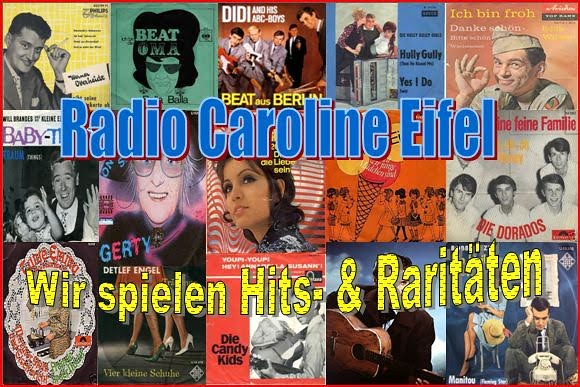This detailed digital poster advertisement for the radio station "Radio Caroline Eiffel" features an assemblage of 15 music album covers, organized neatly into three rows with five covers in each row. The central text "Radio Caroline Eiffel" is prominently displayed at the top in bold blue letters. Beneath this, an additional line of text in yellow reads "Vir Spilen Hitz und Raritäten," suggesting a mix of hits and rarities, likely in German. The collection of album covers behind the text showcases a variety of music genres and artists, ranging from solo performers to bands, including both male and female artists. The entire image is accentuated by a striking red border, tying the composition together and making it visually captivating.